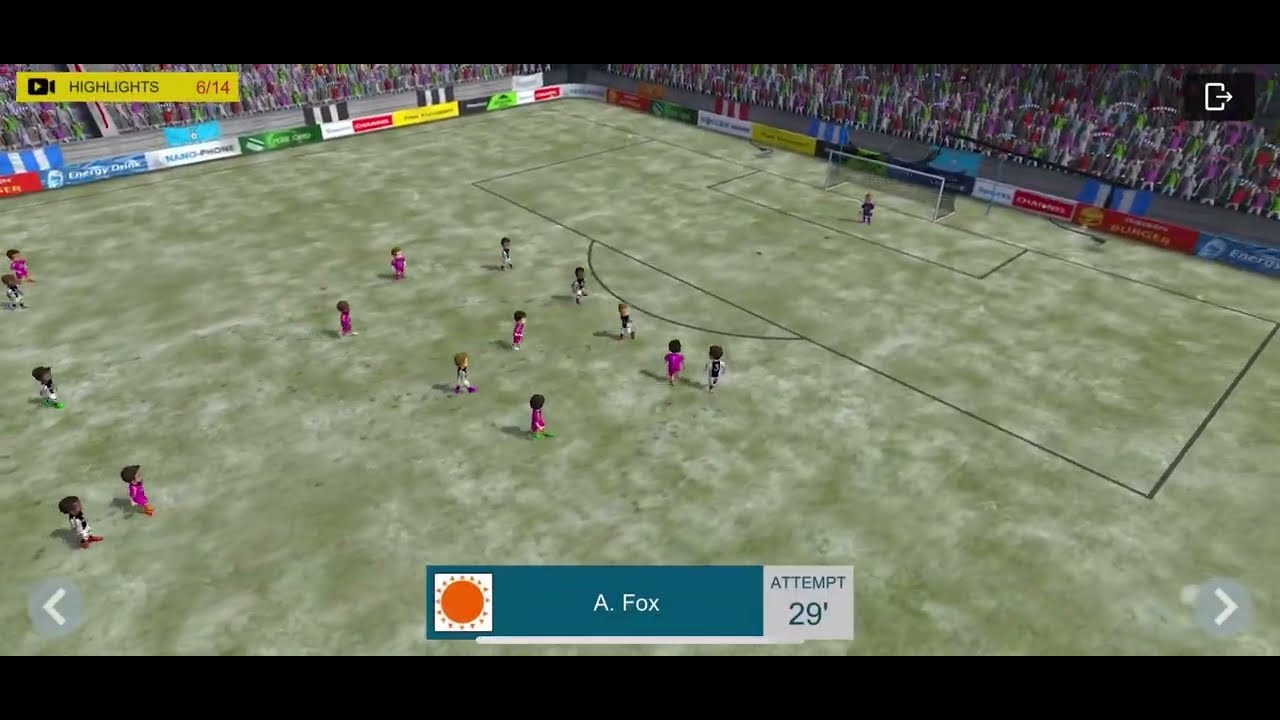The image is an overhead shot, angled downward, capturing a video game scene of a soccer match displayed on a screen, possibly a laptop or TV. The screenshot has letterboxed black borders at the top and bottom, framing the game. The soccer pitch, with its green grass mottled with white patches, occupies the center of the image. Surrounding the pitch is a crowd of blurred, cartoonish spectators sitting in a rectangular formation. To the left of the goal, the stands extend in an L-shape filled with advertising billboards.

Two teams of diminutive, toddler-like cartoon players, dressed in distinct uniforms—one team in black and white, the other in purple—are animatedly running on the field. Only half of the soccer field is visible, with the focus on action near the goal. The bottom of the screen features a banner displaying "A Fox Attempt 29," possibly indicating a game highlight. In the top left corner, a smaller banner with yellow background and text “Highlights” in black and “6-14” in red is visible. A skip-forward arrow icon is situated in the bottom right corner, suggesting control over the video playback.